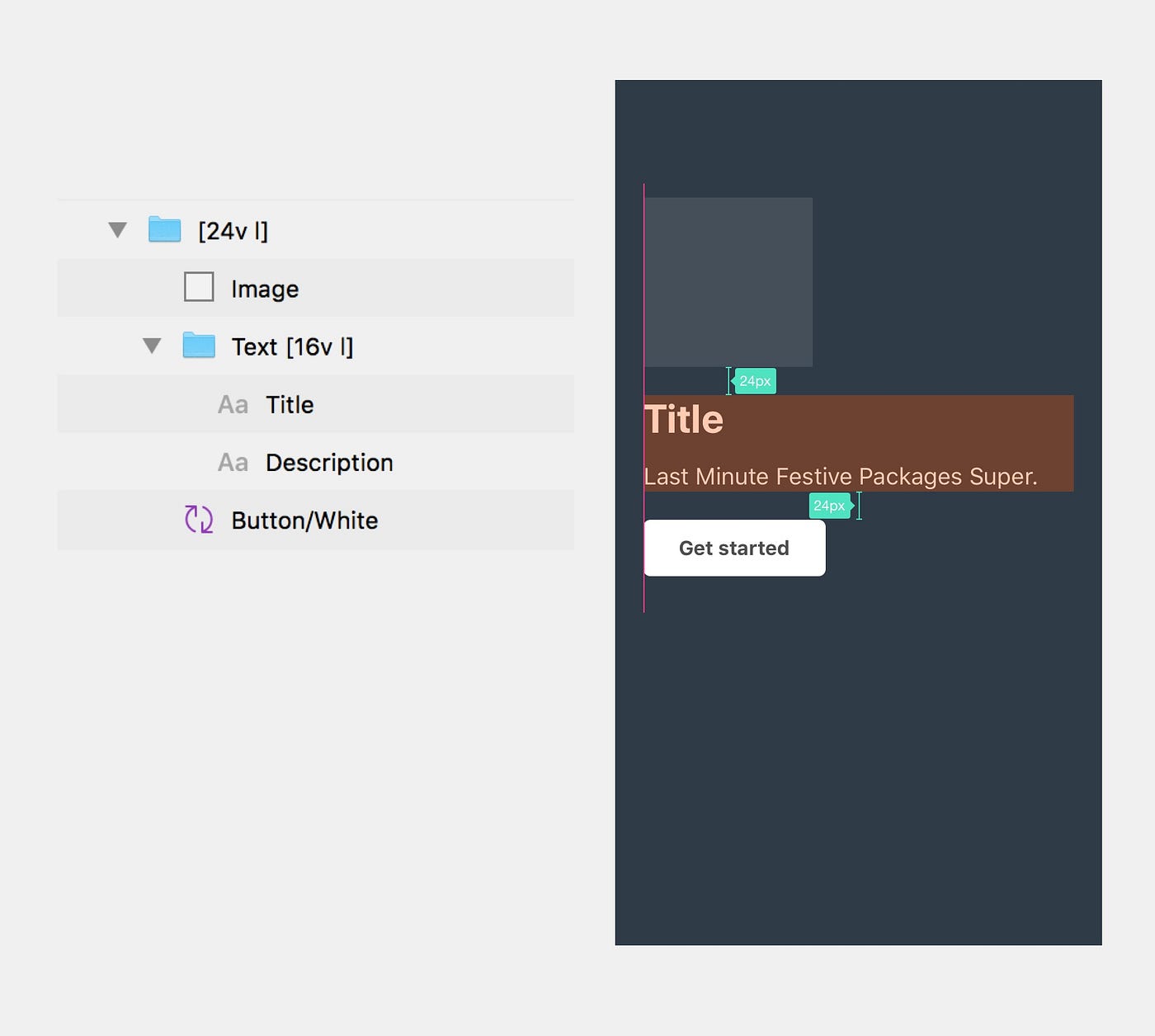A screenshot appears to capture the design interface of an Apple app, likely used for creating a mobile website or mobile app. The left side of the screen showcases various design elements organized in a hierarchical folder structure. The topmost folder, labeled "24VI," possibly indicating the 24th version, contains several sub-elements. Within this, there is an image element followed by a text element marked "16VI" in brackets. Below these, another subgroup labeled "button/white" features a small purple refresh icon next to it. Further down, there are title and description elements, each with a text icon to their left.

The right side of the screenshot displays a mock-up reflecting these elements. The mock-up features a dark blue background. Although the image element is present, the actual image has not been loaded, suggesting its intended placement. There is a 24-pixel border between the placeholder for the image and the title. The title reads "Last-minute festive packages," followed by a period. Below this title, there is another 24-pixel spacing before a "Get Started" button, which is styled with a white background. The text on the button matches the background color of the overall design, maintaining a cohesive visual theme.